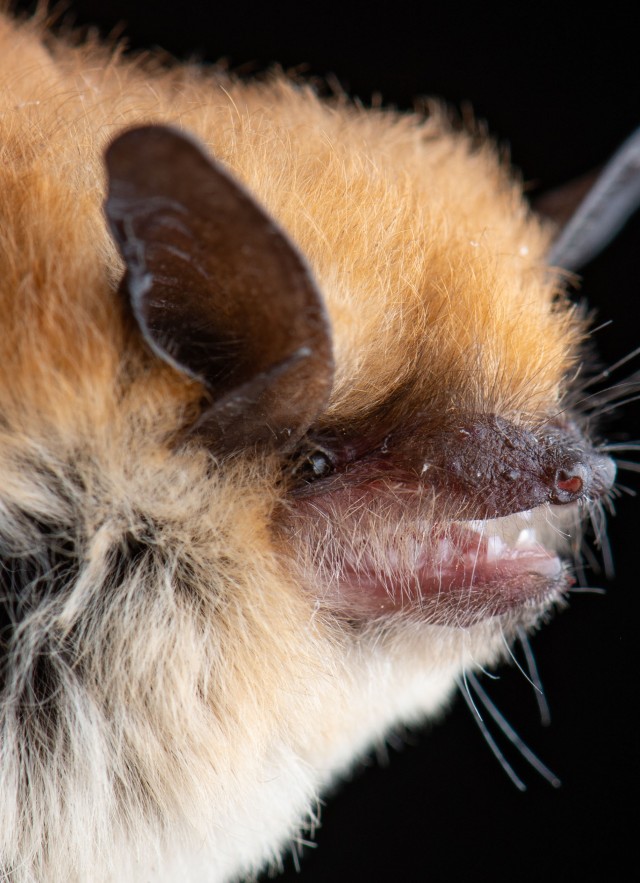This close-up image captures the intricate details of a bat's face set against a solid black background. The bat features a long, dark brown muzzle ending in a rounded nose with a visible pink nostril. Its mouth is ajar, revealing white, sharp teeth and pink gums, partially obscured by yellow whiskers. The bat's dark, black eyes appear sunken towards the back of its head, just below a large dark brown ear that arches upward, curving to the right and back to the left with a slightly jagged edge. The top of its head boasts a tuft of tall, light brown fur, with white fur underscoring it and hints of black skin peeking from beneath. The fur transitions from light brown and tan at the top to white at the lower part of the face. In the upper right corner of the image, there is a suggestion of a wing, possibly in flight, adding to the sense of movement and alertness in the bat.